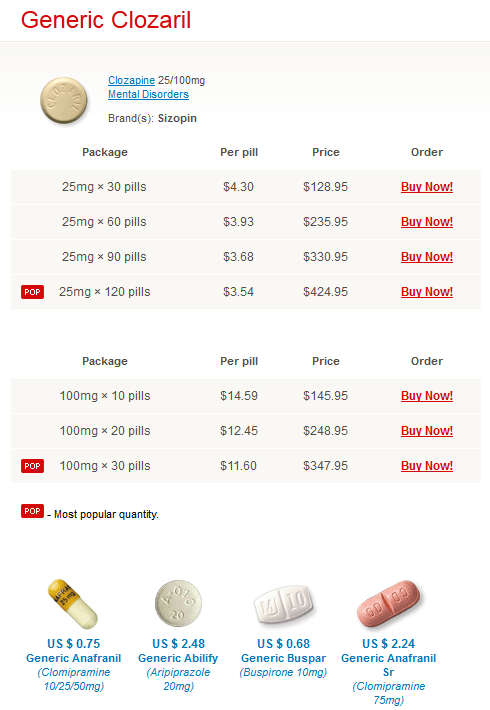The image features a promotional layout for a medication named Clozaril. At the top, the background is white with the word "generic" written in red, followed by the medication name "Clozaril" in large text. The background then transitions to gray, highlighting a beige-colored pill in the foreground.

In blue text, the name Clozaril is repeated along with the dosage information "25/100 mg" in black. Below this, in blue text, the words "mental disorders" are displayed. Further down, "Brand: Sysopin" is specified in black, along with packaging details: "Package: 25 mg x 30 pills," followed by options for 60, 90, and 120 pills. A red rectangle with the word "POP" in white is present, listing per-pill prices as $4.30, $3.93, $3.68, and $3.54, respectively.

The total prices are listed as:
- $128.95 for 30 pills,
- $235.95 for 60 pills,
- $337.95 for 90 pills,
- $424.95 for 120 pills.

Each package option includes a "Buy Now!" button in red, underlined with an exclamation point.

Further down, similar packaging options are presented for 100 mg dosages with 10, 20, and 30-pill counts. The per-pill prices are $14.59, $12.45, and $11.60 respectively, with total prices of:
- $145.95 for 10 pills,
- $248.95 for 20 pills,
- $347.95 for 30 pills.

Each of these options also includes a prominent "Buy Now!" button in red.